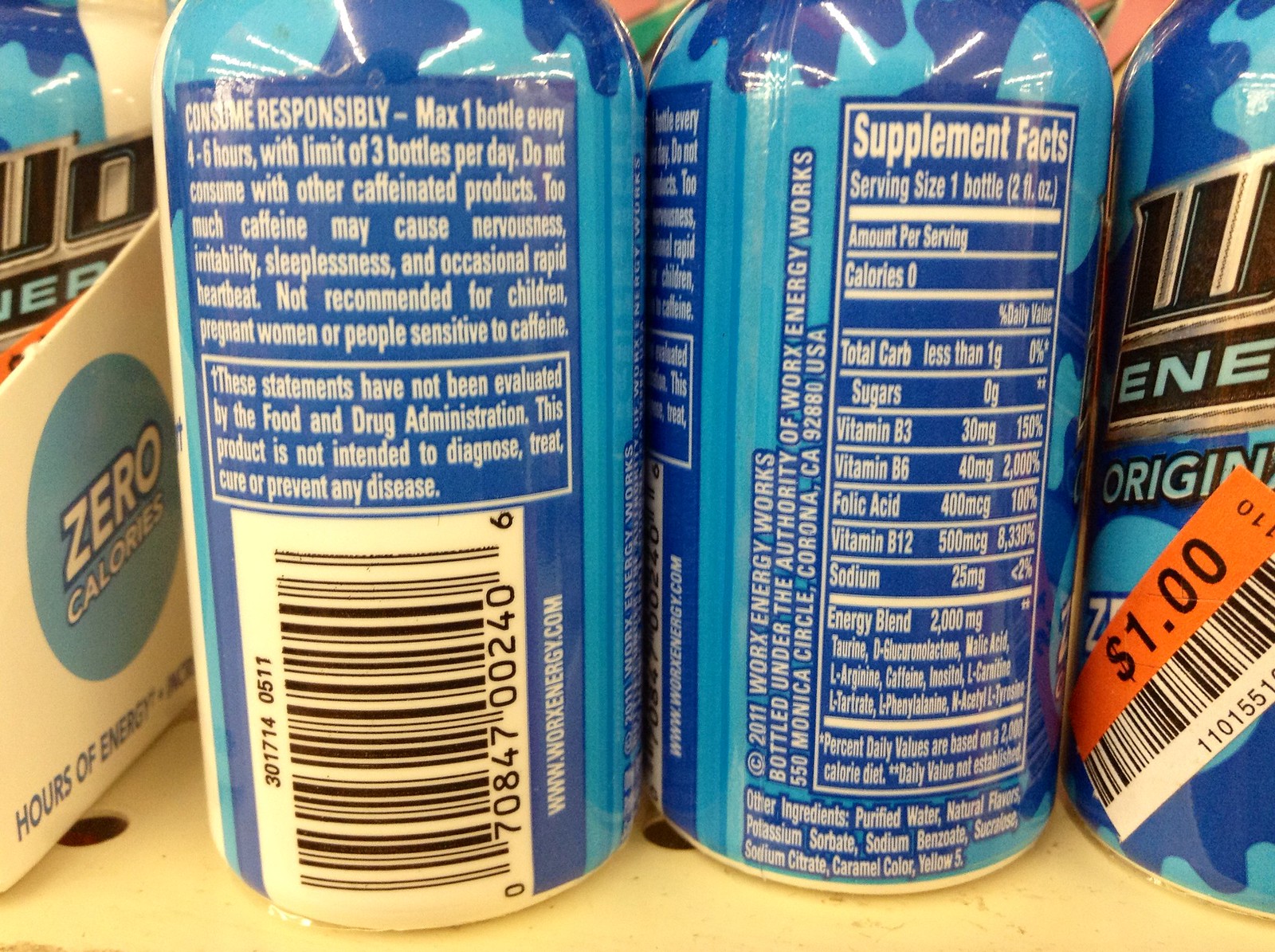The image depicts an extreme close-up of four blue energy drink cans prominently displayed on a cream-colored shelf. The cans, which are "Works Energy" drinks, have dark blue accents and showcase the word "energy" beneath the brand name starting with a 'W.' Supplement facts labels, indicating zero calories, are visible on the side of the cans. Additionally, the cans' nutritional information highlights various vitamins and a "consume responsibly" message. One can on the far right features a clearance sticker with a barcode, stating $1 in bold black font on an orange background. To the left of the cans is a small white cardboard box displaying a logo within a light blue circle, also mentioning "zero calories."